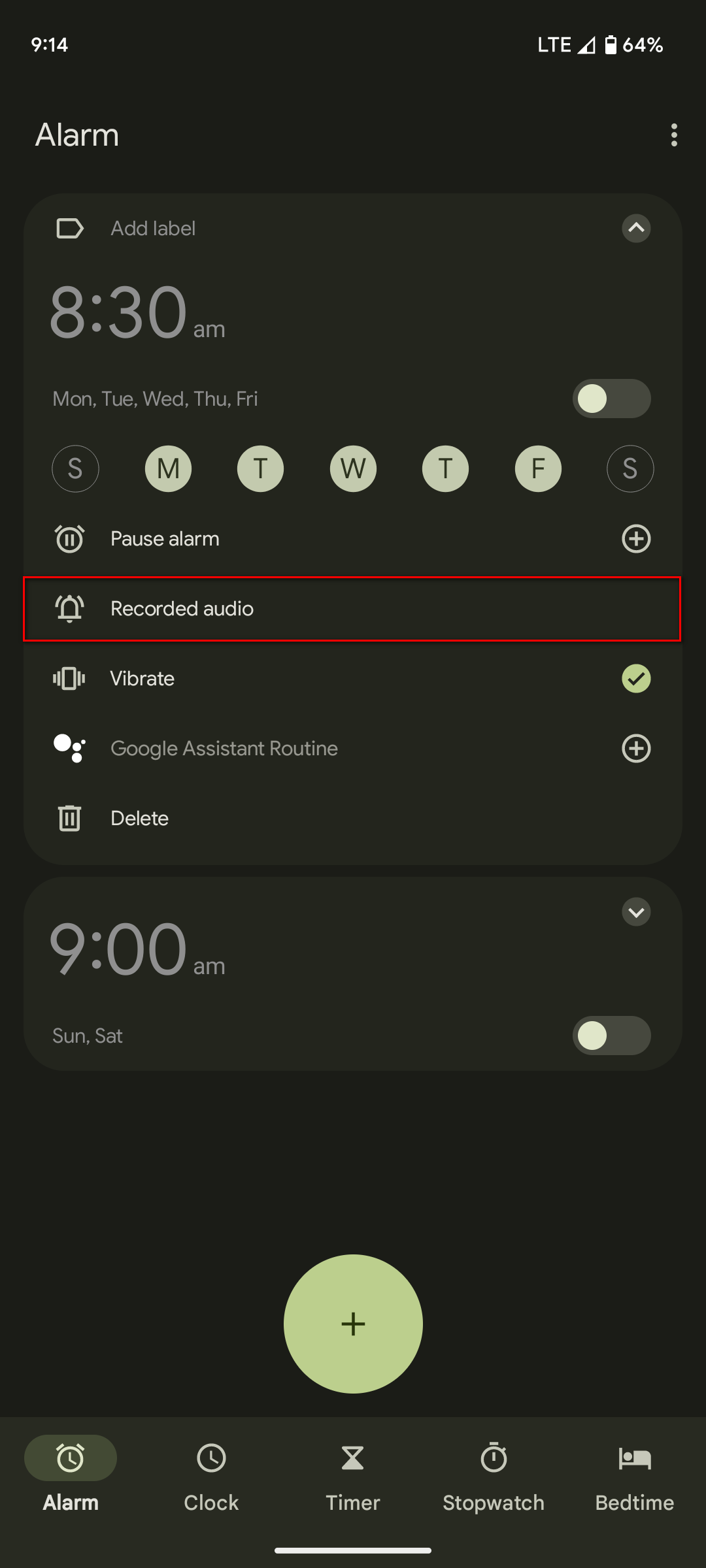This vertical smartphone screenshot primarily features a dark-themed interface with a black background. The screen shows various shades of dark gray boxes, creating a contrast against the backdrop. In the upper left corner, the time is displayed as 9:14. Meanwhile, the upper right corner includes indicators for LTE connectivity, a small triangle icon, and battery life at 64%.

In the central part of the screen, the 'Alarm' label is prominently showcased in white with three vertical dots beside it, indicating more options. Below this, a dark gray box reads 'Add label,' followed by the specifics for an 8:30 AM alarm. The alarm is set but not yet toggled on. The days of the week—Monday through Friday—are listed with the selected days highlighted.

The interface also includes options such as 'Pause alarm,' 'Record audio' (highlighted), 'Vibrate' (checked on), and 'Google Assistant routine,' which has an addition ('+') sign next to it. At the bottom of this section, there is a 'Delete' button and the scheduled times for additional alarms: one for 9 AM, with Saturday and Sunday yet to be toggled on.

At the very bottom, the menu includes options for 'Alarm,' 'Clock,' 'Timer,' 'Stopwatch,' and 'Bedtime,' providing a full suite of time-management tools.